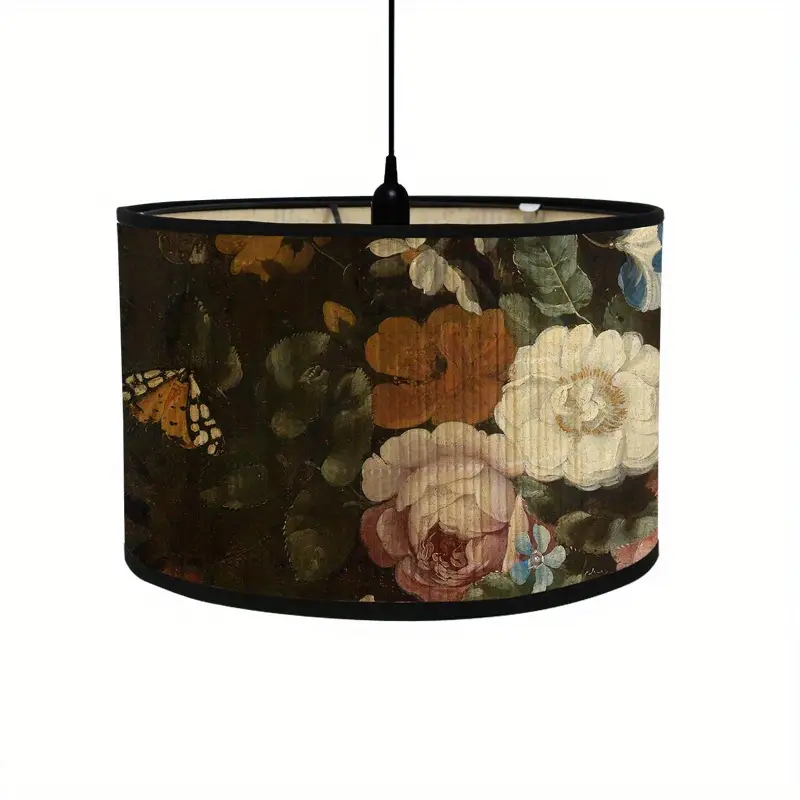This image features a vintage-inspired hanging light fixture, likely from the 60s or 70s, consisting of a single black wire suspending a light bulb. The focal point of this fixture is its cylindrical lampshade, which is open at both the top and bottom and adorned with a vibrant nature-themed design. The lampshade's exterior showcases an array of florals and greenery, including orange, pink, red, white, and blue flowers, possibly roses, camellias, and forget-me-nots, giving it a lush, pastoral appearance. A striking monarch butterfly with yellow and orange wings is also depicted amidst the florals. The cover features a black trim along its edges, with the inside appearing beige. Set against a white background, the scene captures a wildlife aesthetic imbued with rich, dark colors and a touch of fall ambiance, making it a distinct and striking decorative piece.